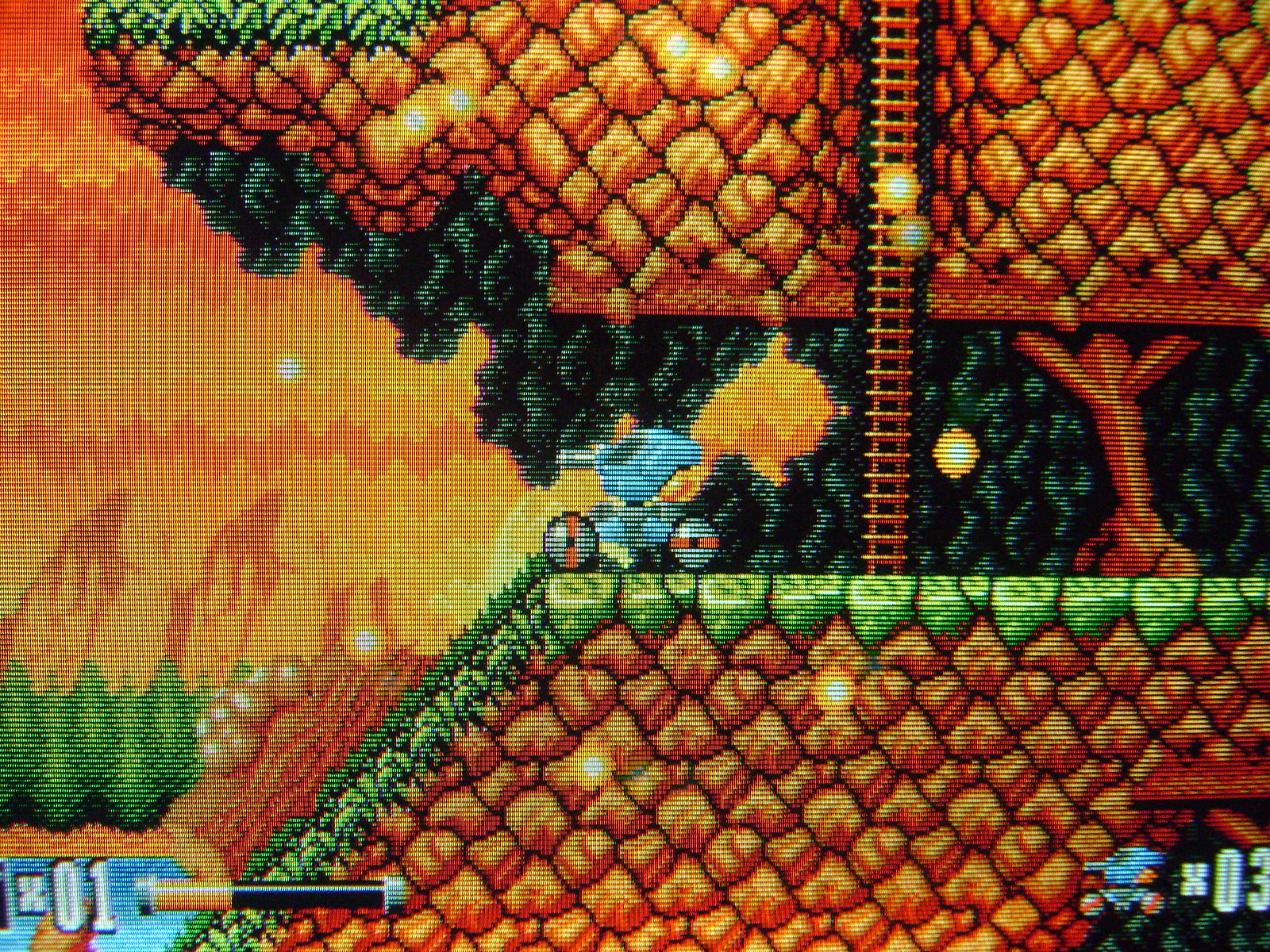The image depicts an old, pixelated 2D video game screenshot with low-resolution graphics and a vivid color scheme dominated by bright orange, red, and yellow hues. It features an orange and yellow sky with dark green or bluish trees in the background. The green platform ascends a rocky landscape dotted with orange and yellow rocks. In the middle of the scene is a central ladder that connects the rocky areas, and there is a tunnel-like structure between them. There is a small blue vehicle-like object with two wheels, which could be robotic, emitting an orange flame as it moves along the ledge between the structures. At the bottom left, the text "Time Zone 1" is displayed in blue, alongside a partially depleted health bar indicating more than half of the power has been used up. The bottom right corner shows "Time 03" with an icon of the blue vehicle, suggesting three lives remaining. The overall static and lined appearance suggests the image was taken from a TV screen or is a capture from a vintage game.